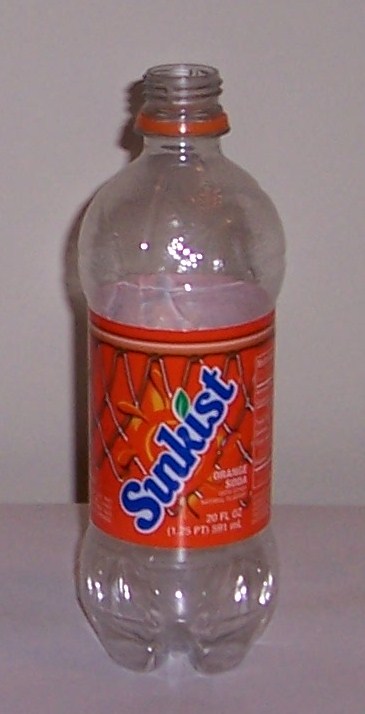This photograph captures an empty, clear plastic bottle of Sunkist orange soda placed on a grayish countertop with a faint shadow cast on a gray wall behind it. The bottle prominently features an orange label encircling its middle, diagonally adorned with the word "Sunkist" in a blue, rounded font. The "i" in "Sunkist" is uniquely dotted with a green leaf. Beneath the brand name, small white text declares "orange soda." The label also includes the volume, noting "20 fluid ounce (1.25 PT)." An orange plastic ring, a remnant of the removed cap, sits at the top of the bottle. The bottle’s base is designed with four small feet, and the entire surface reflects light, creating glares on both its lower and upper portions.